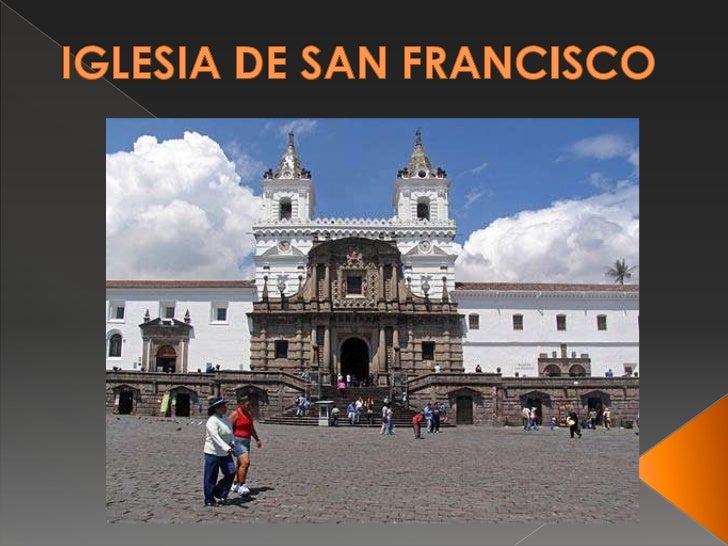The image depicts the picturesque facade of Iglesia de San Francisco, framed by a gray and black border, with 'Iglesia de San Francisco' prominently displayed in capitalized orange letters at the top. The architectural grandeur of the building is highlighted by its predominantly white stone construction, contrasted with rich brown embellishments and featuring intricate decorative stonework. The church features two imposing white towers on either side, each crowned with needle-pointed spires and adorned with windows. 

In front of the church, a broad staircase leads up to the main entrance, surrounded by a bustling courtyard paved with stone pavers. Numerous people, dressed in a variety of outfits, are moving around the area, lending a sense of life and activity to the scene. Among them, two women stand out on the left: one in a red tank top paired with blue shorts and white shoes, and the other in a white long-sleeved shirt, blue pants, and a blue hat. 

The sky overhead is a vibrant blue, filled with large, fluffy white clouds, enhancing the serene atmosphere. A tree, possibly a palm, is visible at the upper right corner of the image, adding a touch of natural beauty to the architectural splendor.